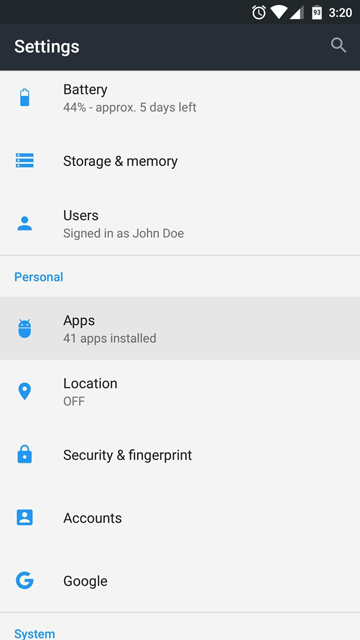The image is a screen capture from a mobile device, displaying the "Settings" menu. The word "Settings" is prominently written in white letters on a dark gray bar at the top of the screen. Below this bar, various settings options are represented by blue icons, aligned vertically along the left side of the interface. 

To the right of the icons, in black text, are the corresponding descriptions:
1. The top icon represents the battery.
2. The second icon pertains to storage and memory.
3. The third icon is associated with user accounts, displaying the active user as "John Doe."

Additionally, the word "Personnel" is highlighted in blue below the user account section. Further down, more blue icons appear, each with their respective descriptions:
- "Apps" next to an app-related icon.
- "Location" followed by a location icon.
- "Security and fingerprint," which is illustrated with a padlock icon.

Each section and icon provides a clear and organized look into the various settings available on the mobile device.